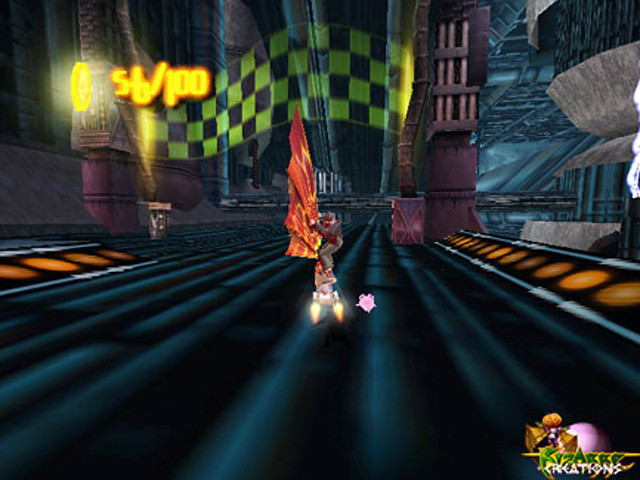This is a screenshot from a fantasy video game. The central character, who is in motion, appears to be riding a futuristic hoverboard with jet flames emitting from the back and holding a red and yellow parasail. The setting features a blue racetrack-like roadway illuminated with lights on its sides. In the bottom right corner of the screen, there's a logo with the words “Bizarre Creations” and an image of a character with a pumpkin head. A green and black checkered flag hangs between two purple columns at the top middle of the screen. The upper left corner displays numbers, possibly 5, 6-100, indicating some form of in-game metric. The flooring displays dark, vertically aligned wires, adding to the futuristic ambiance.